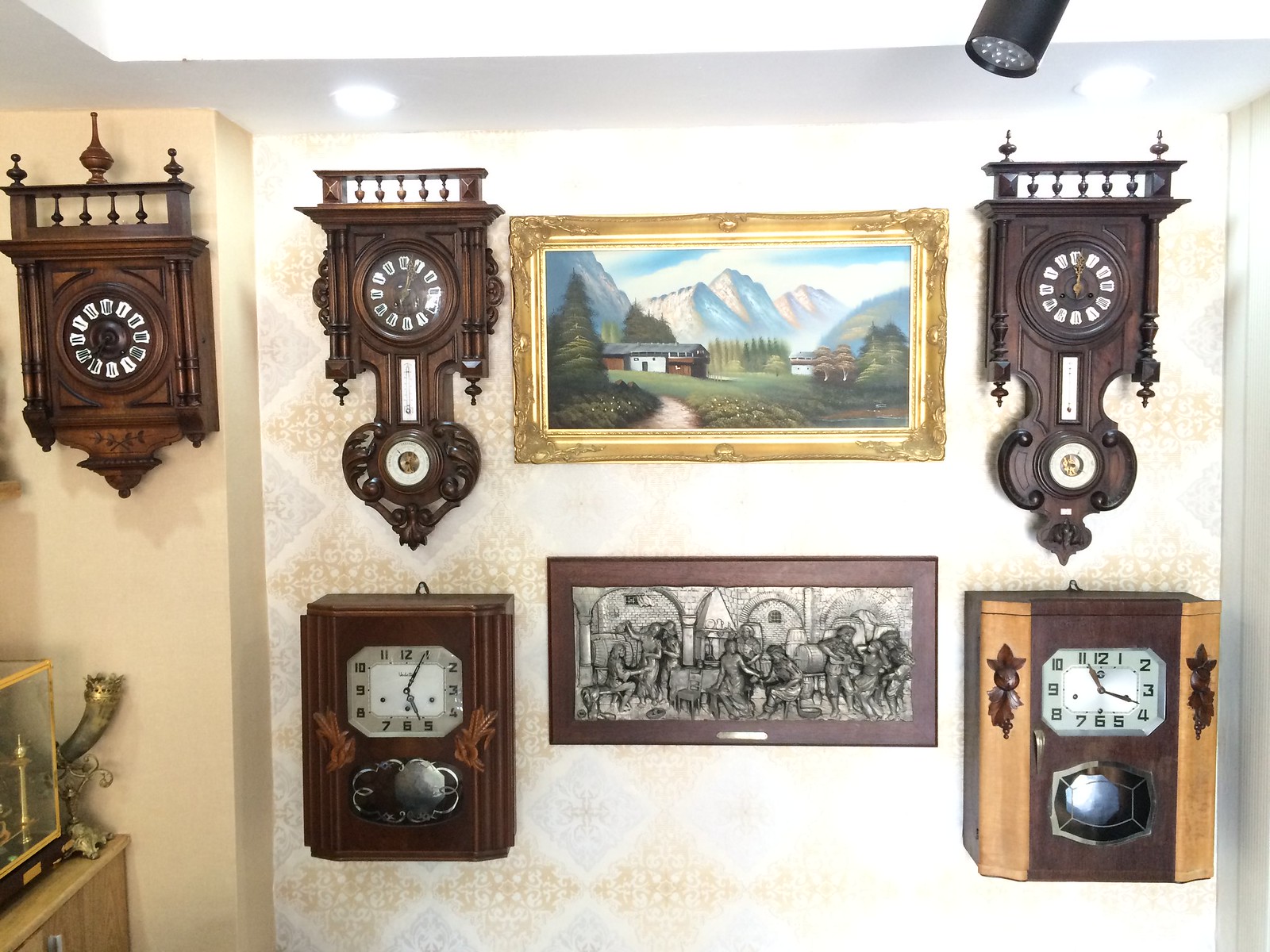This photograph showcases an elegantly decorated light brown wall with a diamond pattern accented by silver diamonds, accompanied by an adjacent orange wall to the left. The white ceiling and bright illumination suggest a display case area. The centerpiece is a collection of five intricately designed, antique-style wooden clocks, each detailed and unique, creating a harmonious yet varied arrangement. The upper left clock features a mostly rectangular shape with ornamental detailing including rails on top and spires with orbs. Adjacent to it, a clock with a square top and a heart-shaped bottom is mirrored on the other side of the wall by a similar clock, though this one ends in a circular bottom. Beneath these, two longer rectangular clocks are positioned, each exhibiting distinct characteristics. Flanked between these antique timepieces are two art pieces positioned centrally with a large gap between them. The upper painting, enclosed in a golden ornate frame, depicts a serene village set against a mountain range with pine trees. Simple yet rustic, the lower black and white painting, in a brown frame with a gold placard, illustrates an indistinct group of figures that might represent peasants. Additionally, a display case with a gold frame and window, adorned by a gold horn-like piece, is positioned in the lower left of the image, adding to the elegance of the showcase.